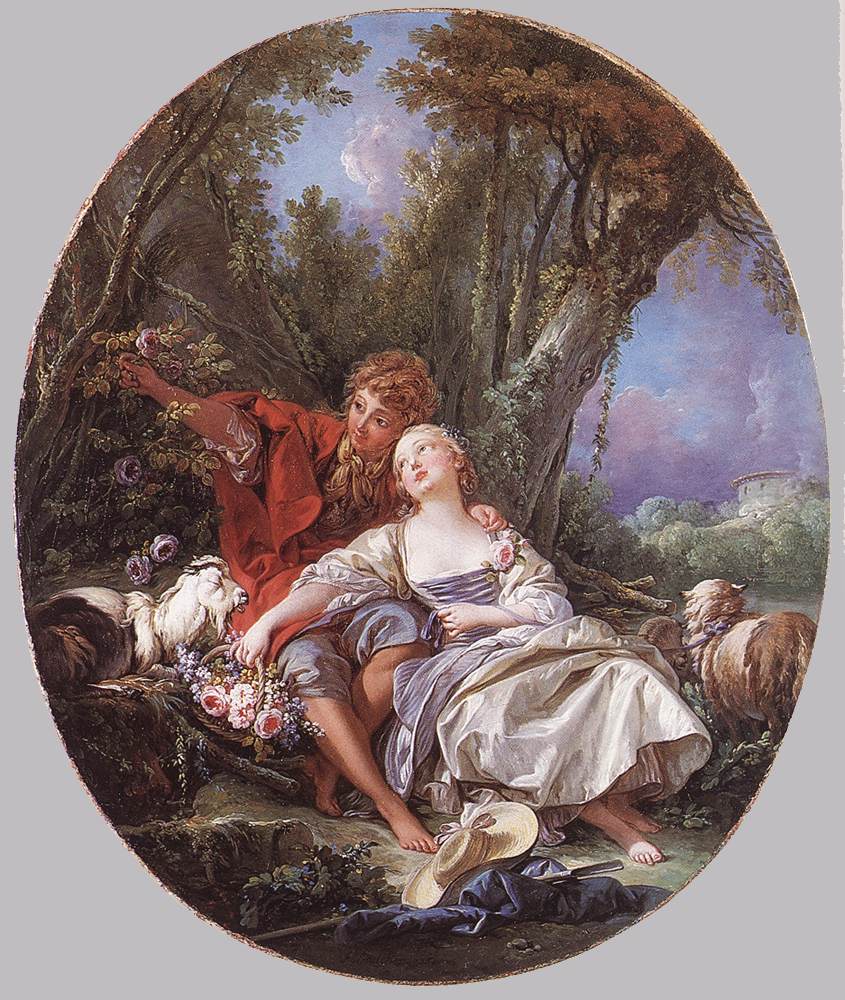This painting, set in an oval frame, beautifully epitomizes the classic Renaissance style, potentially a contemporary piece with an aged appearance. Dominating the scene are a young man and woman, centrally positioned amidst a serene forest backdrop. The man, adorned in a striking red jacket paired with a gold scarf around his neck, sits under a tall tree while picking a flower that hangs just over his shoulder. Beside him, the woman, dressed in a period summer dress, reclines slightly against him with her arm over his lap, holding a basket filled with colorful blooms in her right hand. Nearby, a small goat sits to his left, with a couple of sheep grazing to his right.

Lying on the ground at their feet are a hat and a blanket, adding to the idyllic pastoral setting. Behind them, in the distant background, the hint of a castle structure can be discerned through the foliage, adding a sense of depth and mystery to the scene. The entire composition brings together hues of red, blue, white, gray, and green, creating a harmonious blend of colors that enhance the painting's timeless and romantic quality.